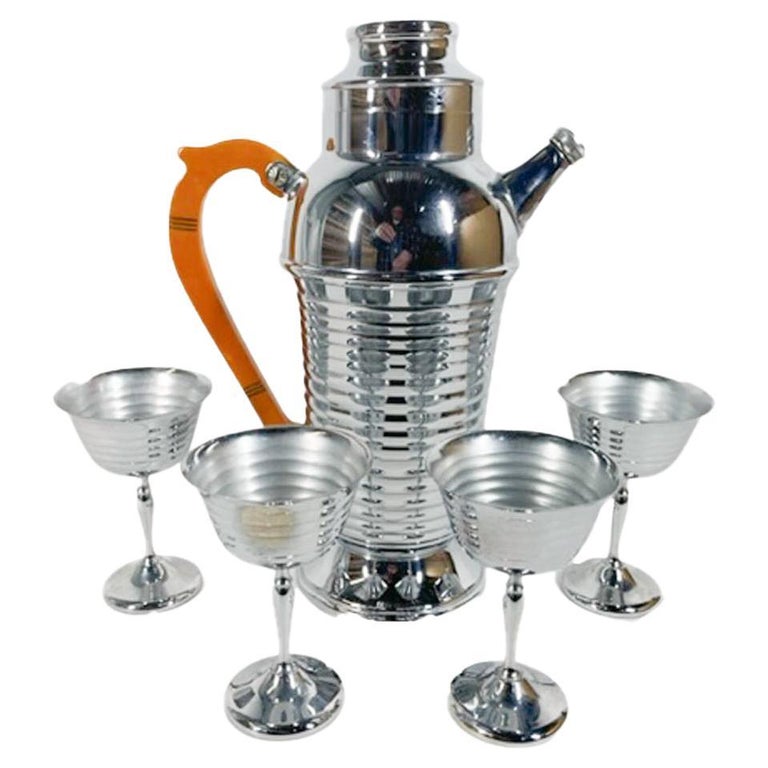The image displays a polished stainless steel or aluminum teapot with a distinctive orange handle, accompanied by four matching long-stemmed drinking glasses. The set is intricately designed with delicate lines and circles that echo throughout both the teapot and the glasses. The glasses are empty, indicating either a ready-to-serve setting or a display. The entire ensemble is placed against a pristine white backdrop. Notably, the reflection of the photographer, an older man wearing a blue plaid shirt with white lines, is clearly visible on the highly reflective surfaces of the teapot and glasses. He is capturing the image with an iPhone, adding an element of human presence to this otherwise static arrangement. The teapot has a removable lid, hinting at its functionality amidst its display.